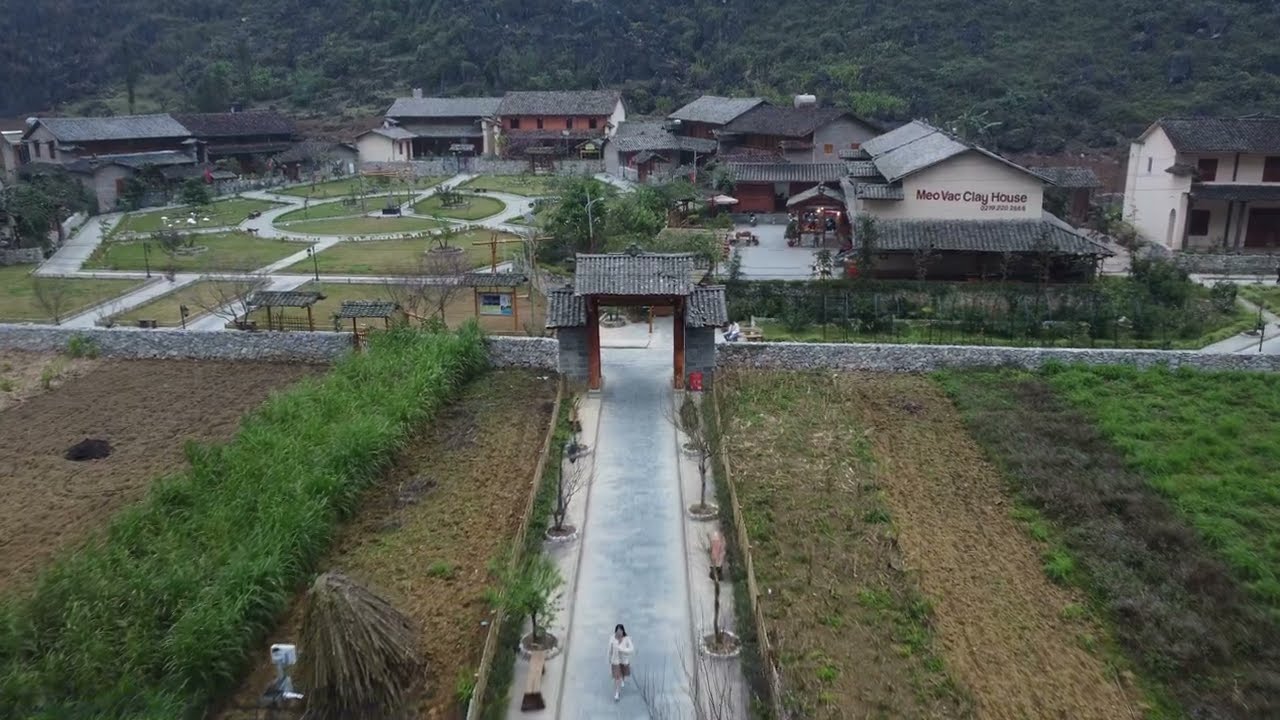This aerial photograph showcases an organized semi-circular arrangement of buildings and a central garden area. The garden, positioned at the heart of this complex, is lush and green, featuring a circular or hexagonal shape bordered by a distinctive white pathway. Encircling the entire area is a green stone wall accented with metallic fencing. A prominent gateway intersects the boundary wall, leading to a blueish walking path flanked by trees. 

Walking along this path is a woman dressed in a white sweater and either a skirt or shorts. To either side of the path are open fields with scattered bushes and some cultivated plants. Nestled in this organized layout of structures, one of the buildings bears the inscription "Meovac Clay House," indicative of the area's blend of residential or possibly resort-like purposes.

In the background, beyond the buildings and garden area, lies a hilly terrain densely covered with trees, adding a natural contrast to the structured environment below. The hills are partially visible, extending upwards out of the frame. The overall setting suggests a serene and thoughtfully organized space merging natural and constructed elements, with various tans, browns, and grays of the buildings juxtaposed with the greens of the vegetation and the blues of the central walkway.